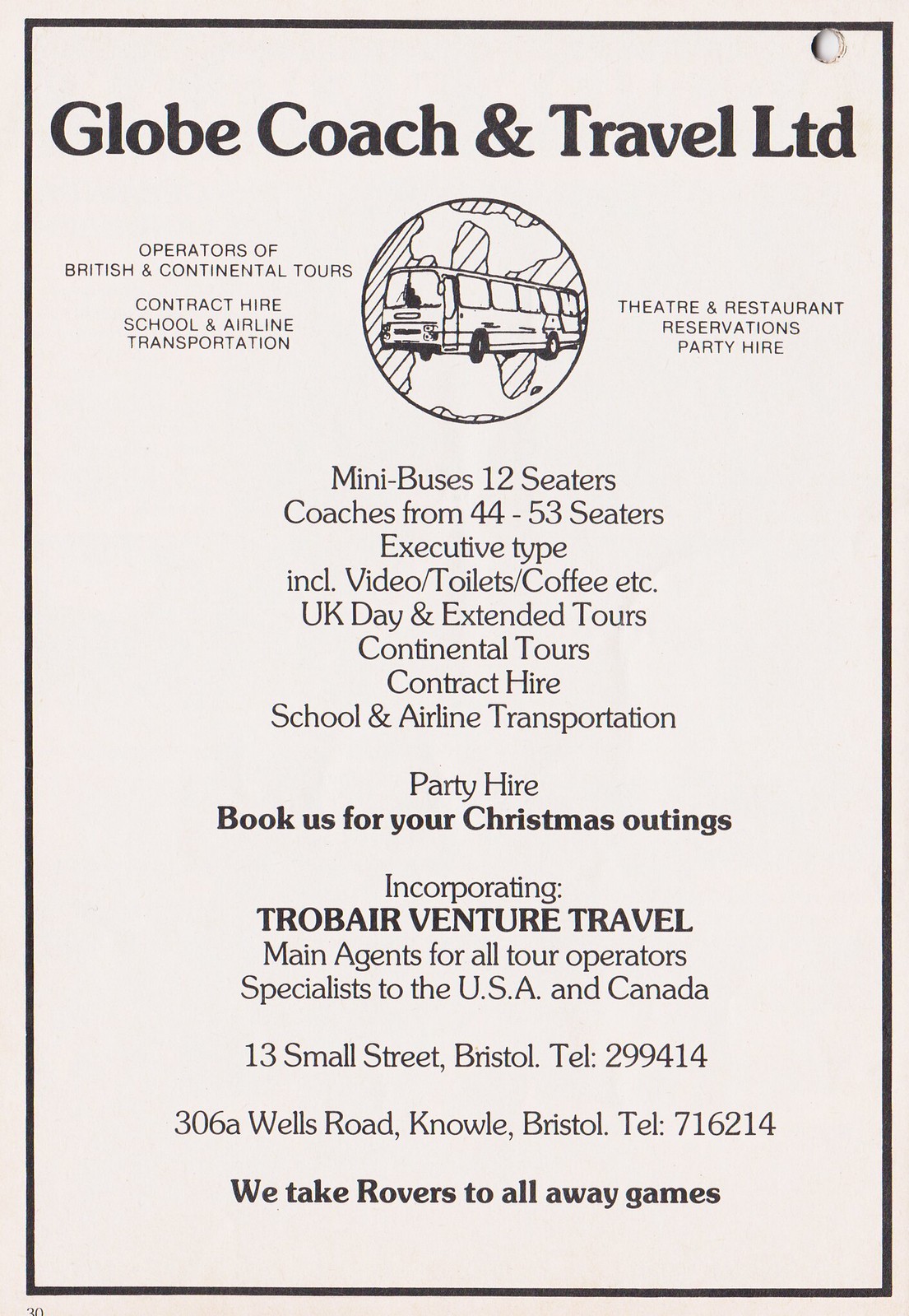This full-page advertisement, likely from a magazine or pamphlet, promotes "Globe Coach and Travel Limited." At the top, it features their name alongside a depiction of a coach bus superimposed on a globe. The ad highlights their services: operators of British and continental tours, contract hire, school and airline transportation, theater and restaurant reservations, and party hire. They offer a variety of vehicles including minibuses (12-seaters) and coaches accommodating 44 to 53 passengers, available in executive types that include amenities like video, toilets, and coffee. The advertisement lists their offerings: UK day and extended tours, continental tours, contract hires, school and airline transportation, and special party hire services, encouraging customers to book for Christmas outings. The ad also mentions their incorporation of Trobear Venture Travel, their status as main agents for all tour operators, and specialists in travel to the USA and Canada. It provides contact details for their offices at 13 Small Street, Bristol, and 306A Wells Road, Knoll, Bristol. At the bottom, it emphasizes, "We take rovers to all away games." The page number 30 is visible at the very bottom.